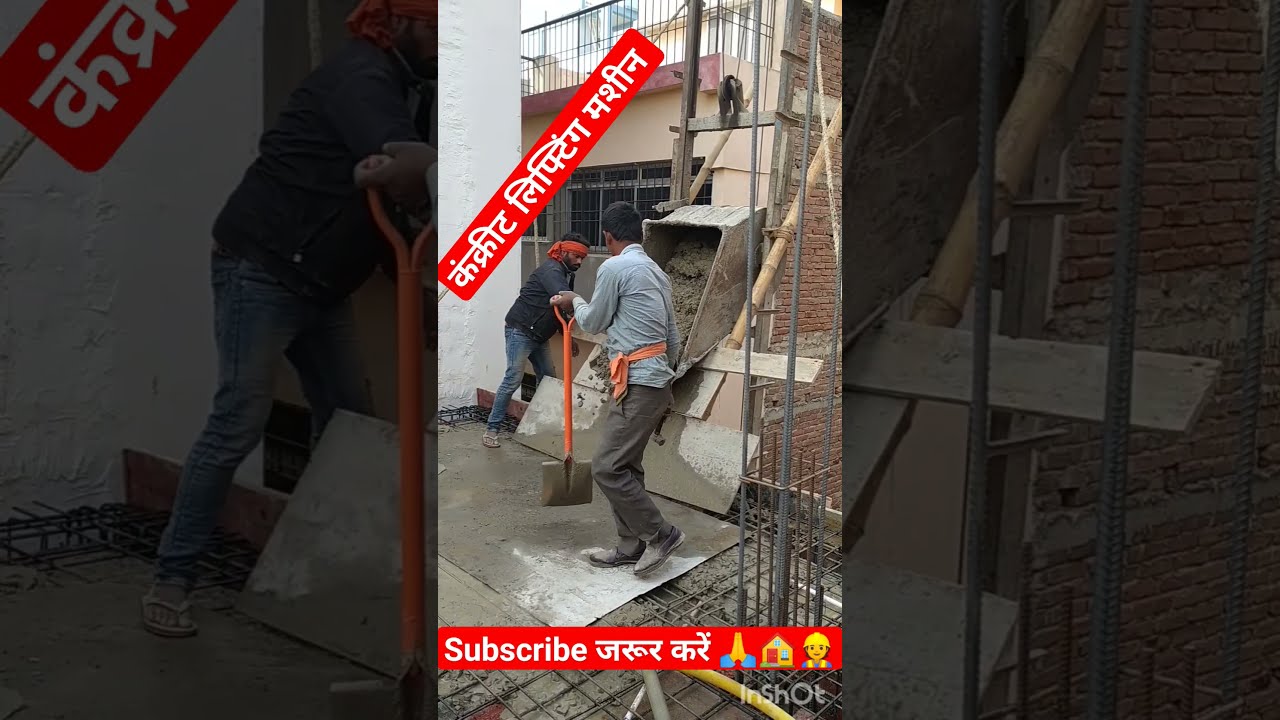This image depicts two Indian construction workers actively engaged in shoveling concrete on a construction site. The central figure, dressed in a dark blue shirt and gray pants, stands with his back partially towards the viewer, wielding a shovel with an orange and gray handle. To his left, another man, donned in a deep navy blue shirt, denim jeans, and an orange bandana, is also working with concrete. The scene is set against the backdrop of a tall red brick wall and features a chute on the right-hand side, pouring concrete onto the rebar-strewn floor. Above the workers is a structure resembling a building with fencing or a gate. The predominant colors in the image include various shades of gray, blue, orange, red, black, white, and tan. The image also exhibits red captions with white Hindi text, and at the bottom, the word "subscribe" accompanied by emojis of praying hands, a house, and a construction worker. Additionally, a watermark reading "in shot" can be seen. The entire composition suggests that this image might be a screenshot taken from a mobile app like TikTok.